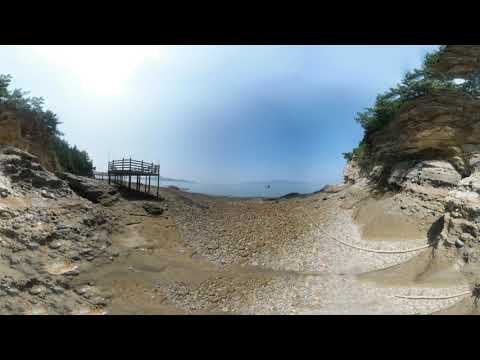This outdoor image depicts a rugged, rocky dirt area leading down to a body of water, framed by cliffs and hills. Dominating the right side of the photo is a steep incline of light-gray rock at the base, which darkens as it ascends and is topped with sparse trees and brush. In stark contrast, the left side features the top of another cliff with greenery and a wooden observation deck elevated on posts, offering a scenic viewpoint. The center of the image showcases a gravelly dirt path, uneven and slightly sloping, guiding the eye toward the distant, serene water. The sky is a clear blue, merging with a lighter hue toward the top left, suggestive of the sun's presence. The overall scene captures a natural, tranquil landscape with a mix of rugged terrain and open vistas.